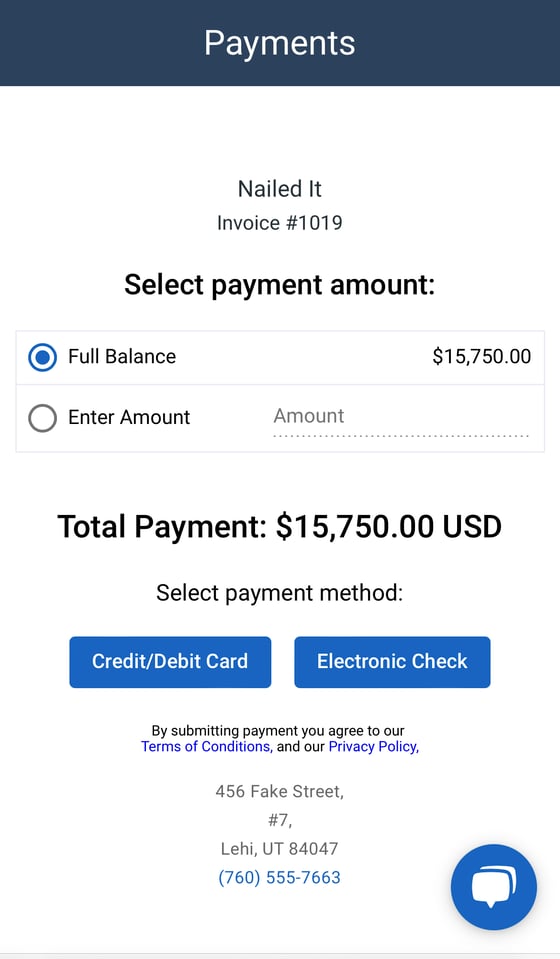Screenshot of a Payment Page:

The image captures a screenshot of a payments page from a website, possibly called "Nailed It," featuring a predominantly white background. At the top of the page, there's a dark blue banner with the word "Payments" displayed prominently in white text. Directly below, in smaller black text, it reads "Nailed It," likely indicating the name of the business.

Below this header, the page displays an invoice number, "Invoice 1019," and prompts the user to "Select Payment Amount." Two radial buttons are presented for payment options. The first button, labeled "Full Balance," is selected and shows a total of $15,750. The second option, "Enter Amount," allows the user to input a different payment amount if desired. 

Continuing down, the page shows "Total Payment" currently set to $15,750 USD. This is followed by a section titled "Select Payment Method," offering two choices in blue buttons: "Credit/Debit Card" and "Electronic Check." 

Below the payment methods, there is a statement in black text: "By submitting payment, you agree to our Terms of Conditions and our Privacy Policy," with both terms highlighted in blue as clickable links. 

Finally, the business's address is listed as "456 Fake Street, Suite 7, Lehi, Utah," along with a contact phone number. Additionally, a small blue button featuring a chat icon is available, presumably allowing users to initiate a live chat for support.